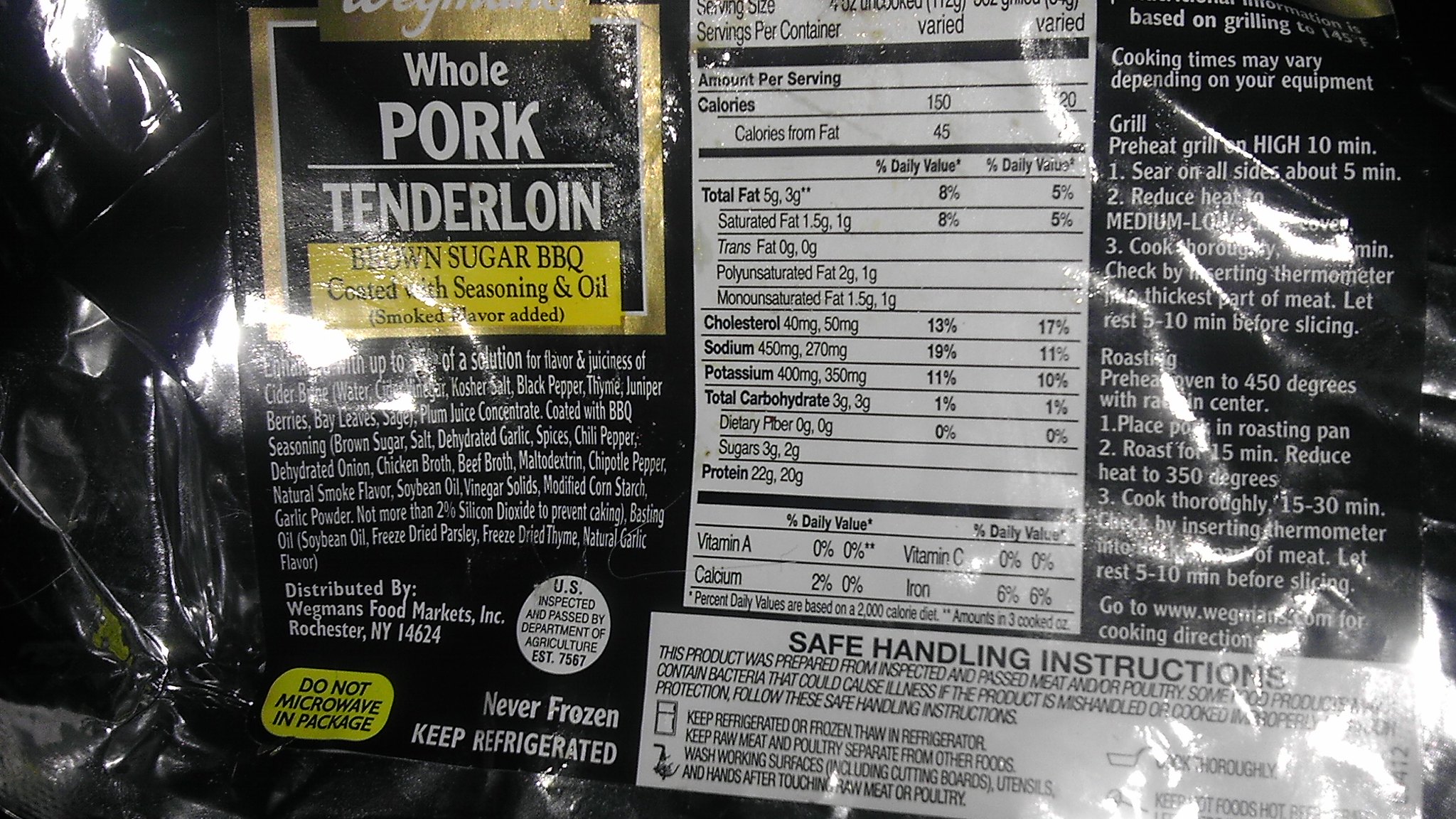This photograph captures the back of a package of whole pork tenderloin encased in a transparent, cellophane-like plastic wrap. The main label is predominantly black with white and yellow detailing. Prominently displayed in white text are the words "Whole Pork Tenderloin," while below that, a yellow bar reads "Brown Sugar Barbecue." This indicates the pork is coated with seasoning and oil with added smoke flavor.

Further details include cooking instructions—grilling, roasting, or general cooking—written in white text on the left side. Adjacent to these instructions, a white box lists the nutritional facts, though the upper part of this box starts midway, with "SERVING" partially visible. Below the yellow text bar, there’s expounded information about the tenderloin being never frozen, requiring refrigeration, and advice against microwaving the package.

Distributed by Wegmans Food Markets Inc., located in Rochester, New York, 14624, this text encapsulates necessary distributor information. The overall design harmonizes black, white, and yellow elements to make key details stand out, ensuring the consumer can easily find and understand the product's specifics.